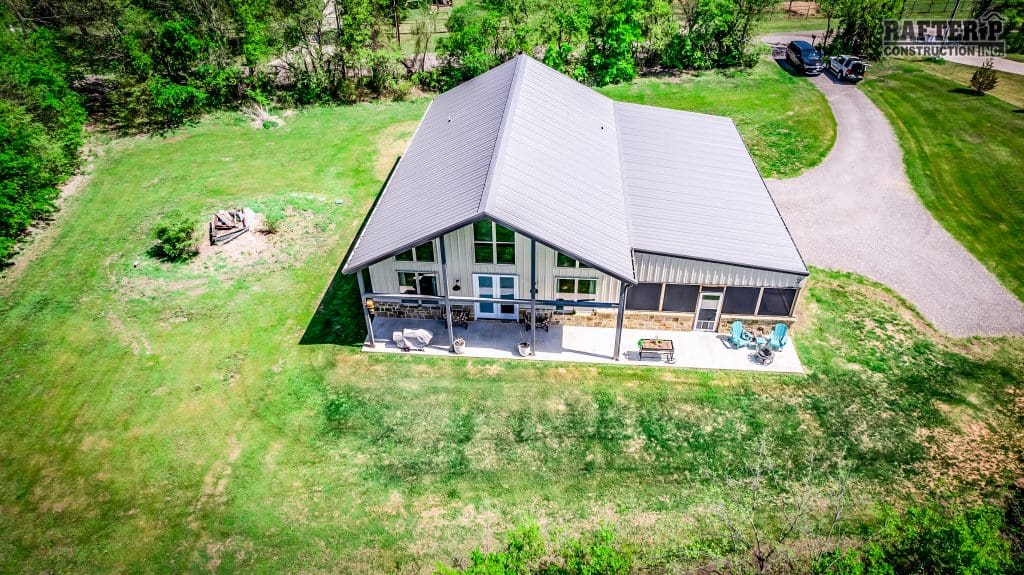The image shows an aerial view of a two-story barndominium with a light gray, fairly flat roof transitioning to a more pitched V-shaped design, especially over the domicile section. The structure includes a utilitarian entrance and a screened porch add-on with white framing. The exterior features white vertical siding and large picture windows at the front and side. The property is set amidst a sprawling green yard with some bare patches, surrounded by a privacy border of trees. In front, there’s a concrete walkway running the length of the house which includes a covered porch area supported by steel beams, furnished with chairs and items for outdoor activities. A curved driveway leads to a T-section near the house, providing ample space for parking, where currently a van and a Jeep are visible. The overall setting suggests a secluded, rural location with no neighboring houses in close proximity.